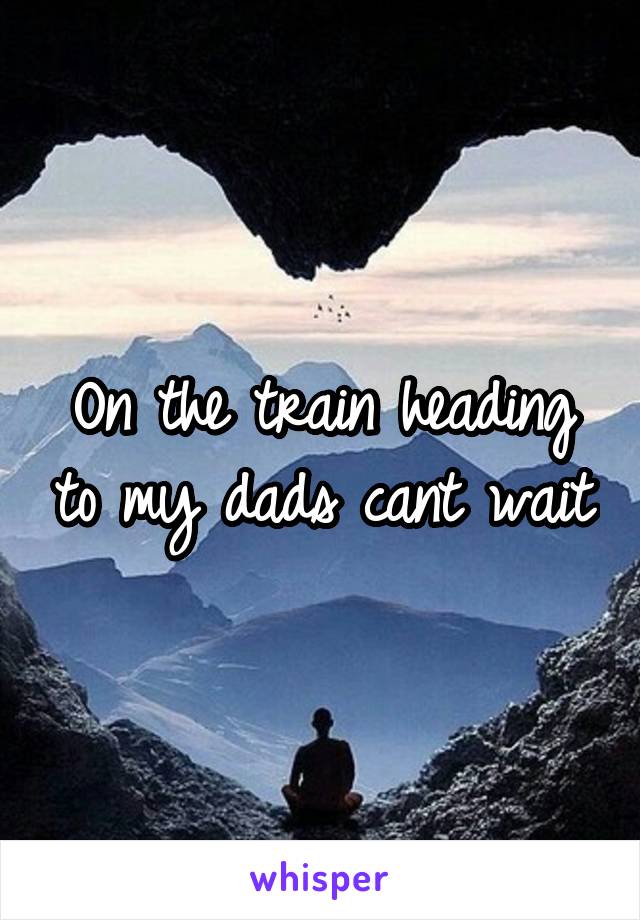The photograph captures a serene scene where a monk, possibly a Buddhist, sits cross-legged and silhouetted in meditation on the edge of a mountain cave, gazing out at a vast expanse of mountains and valleys bathed in a light blue hue. The cave's opening, intriguingly shaped like a heart, frames the picturesque landscape, and the sky, tinged with a reddish hue, suggests the tranquility of evening time. Birds can be seen flying in the sky, adding a touch of liveliness to the tranquil vista. The back of the monk is visible to the viewer, emphasizing his contemplative solitude. In the center of the image, white cursive text with a black boundary reads, "On the train heading to my dad's, can't wait." At the bottom center of the image, the word "Whisper" is displayed in purple text.